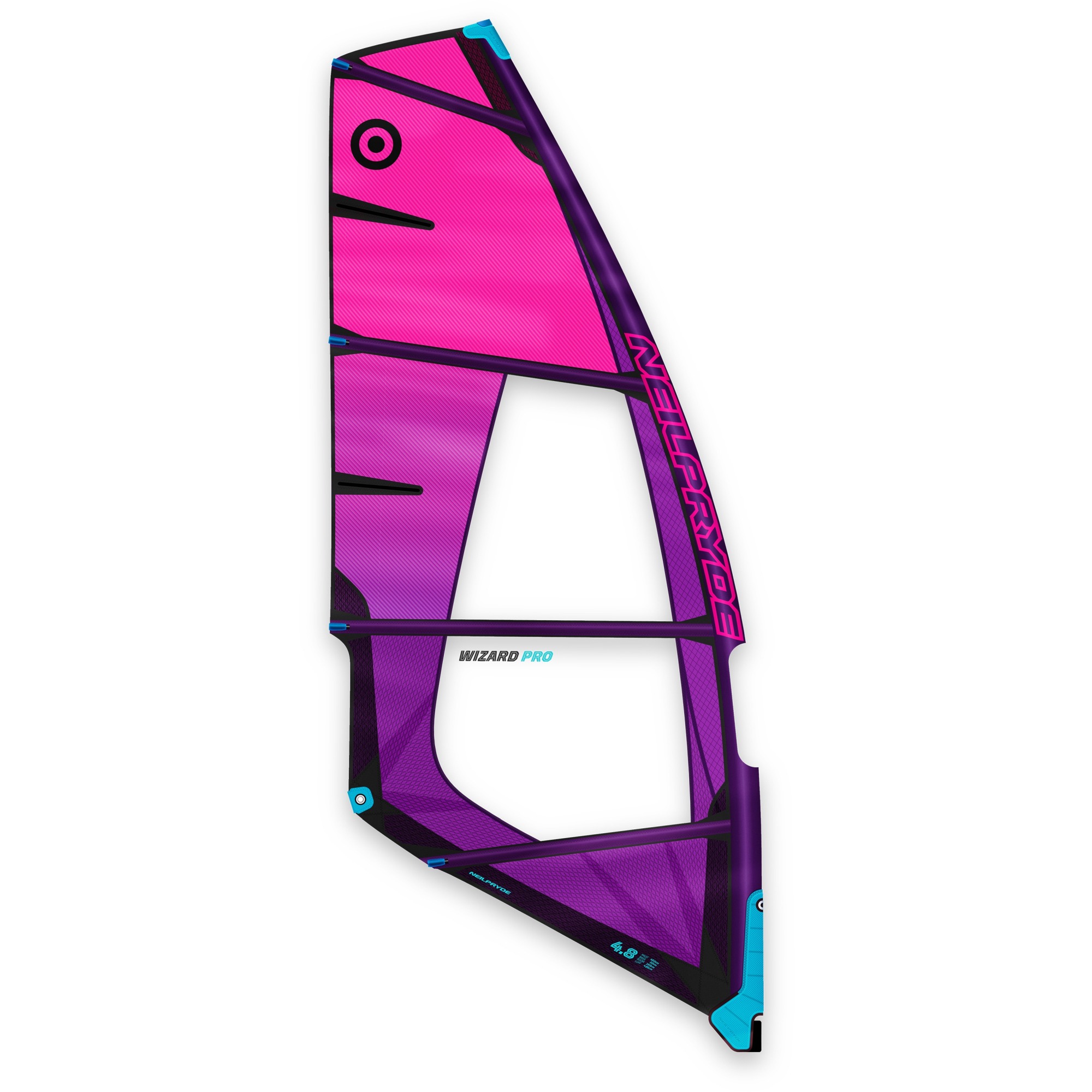The image showcases a vibrant, multi-colored race sail, prominently designed for a sailboard, often associated with windsurfing. The sail dominates the frame with no visible borders, set against a pure white background. Its shape resembles a wing or a curved bow with flowing lines that extend upward from the lower right to the upper left. The sail features a gradient of colors transitioning from bright neon pink at the top to a rich purple at the base, with additional subtle blue highlights along the edges. The sail is adorned with various texts: "Neal Pryde" in neon pink letters against a deep purple backdrop, "Wizard" in black, and "Pro" in light blue. There's also a small, detailed marking that reads "4.6" or "4.8." A distinct clear plastic window in the middle allows visibility for the user when navigating. The overall design is streamlined for performance, indicated by its beam and contours, making it both a functional tool and a visually striking piece of equipment.